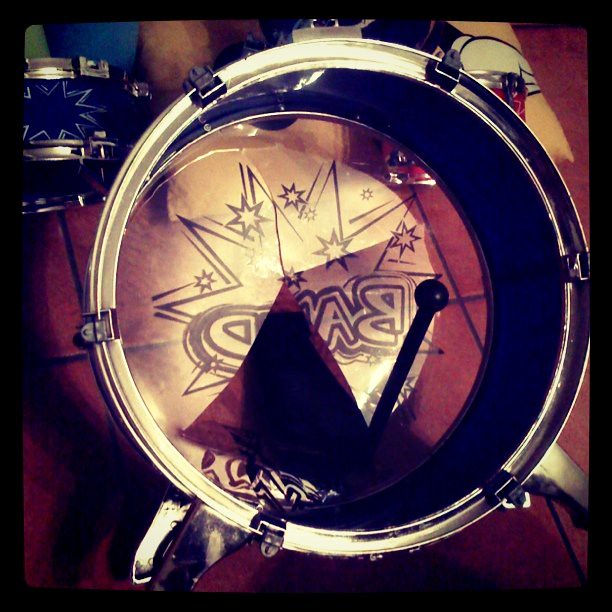The image depicts a bass drum, possibly viewed from either its front or back side, standing upright with a visible black mallet positioned in the middle. The drum features a silver outer rim and legs, suggesting stability, and the drum surface appears clear with writing seen in reverse, indicating the presence of text on the opposite side. The text appears to spell out "BAND" in bubble letters, surrounded by star decorations. 

In the background, there is another drum—a snare drum—characterized by a blue base and silver rims on both top and bottom, adorned with a star design. The setting includes a predominantly red-tiled floor with distinct dark grout lines. Additionally, a small portion of someone's skin, possibly a knee or part of their body, is visible at the top of the image, providing a slight human element to the scene.